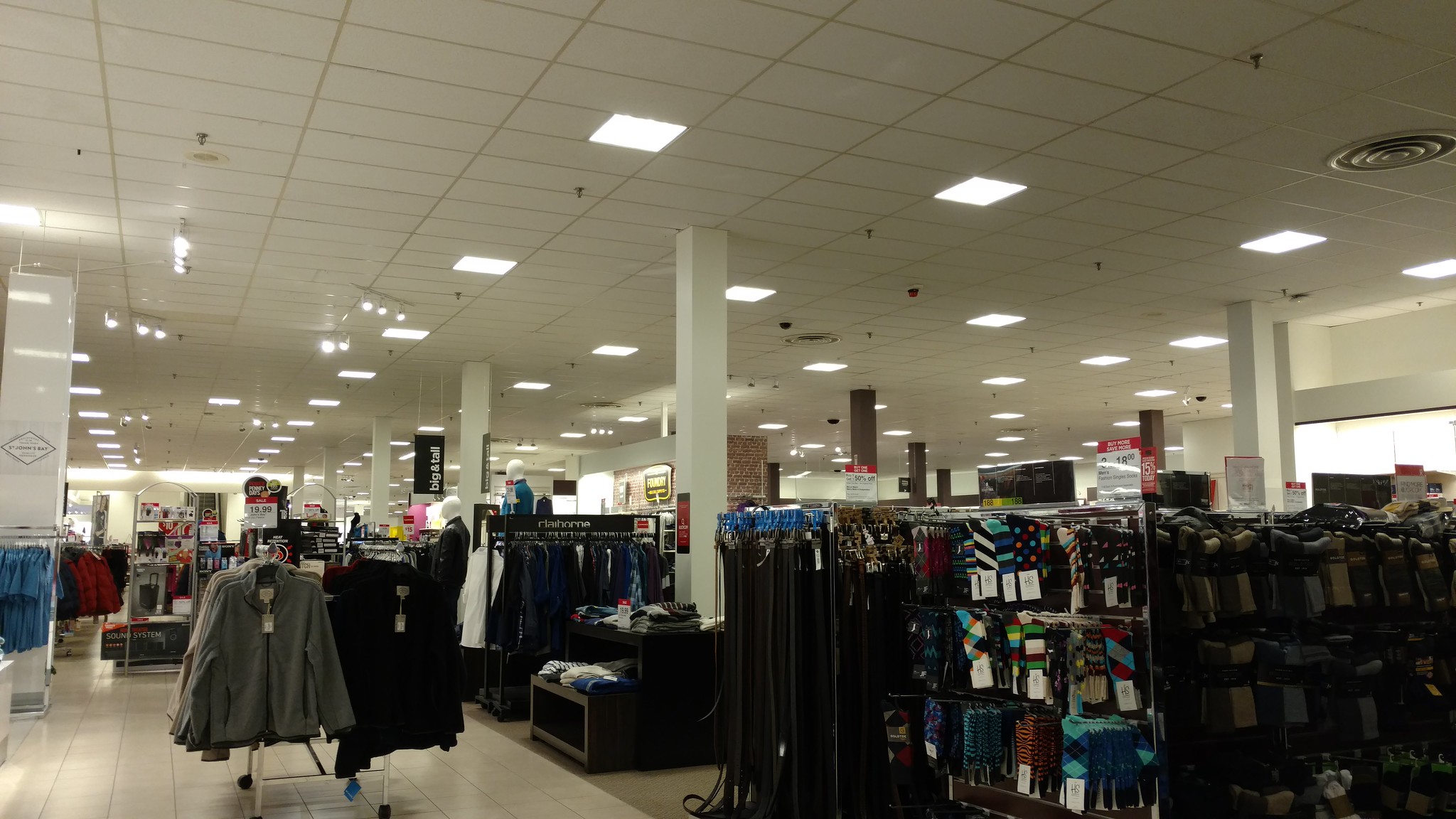The image showcases the interior of a bustling department store characterized by its modern and organized layout. The ceiling is adorned with uniform white tiles, interspersed with large, square fluorescent lights that illuminate the space evenly. Strategically placed metal poles run down the center of the store, providing structural support as well as guiding the flow of shoppers.

In the middle of the store, a prominent display features a variety of clothing items. One rack is prominently filled with an assortment of jackets, complemented by pants or skirts hanging below. Towards the end of this display, a dedicated rack showcases a collection of stylish belts, neatly arranged for easy browsing. Close by, a large rack teems with an extensive selection of socks, ensuring a wide range of choices for customers.

Mannequins positioned along the aisle are dressed in eye-catching blue outfits, adding a splash of color and style to the scene. Adjacent to these mannequins, another rack is filled with blue shirts, meticulously organized. Nearby, a separate rack displays a vibrant array of red shirts, offering additional options for fashion enthusiasts. The overall atmosphere is one of orderliness and variety, inviting shoppers to explore the diverse offerings available.